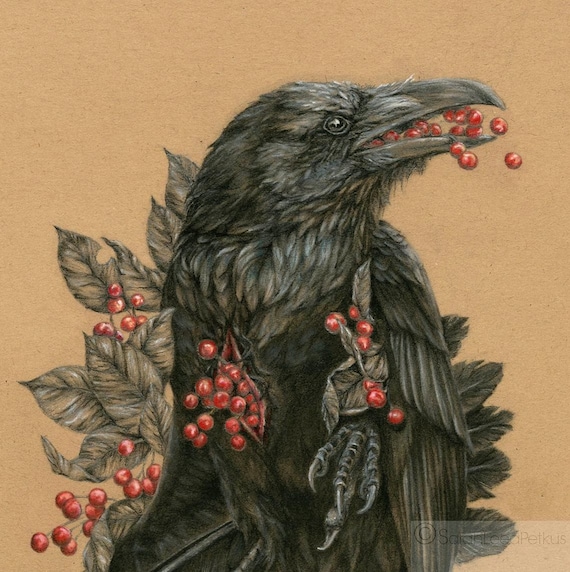This highly detailed illustration features a blackish-brown crow surrounded by dark foliage, set against a sepia-toned, brownish-red background reminiscent of textured cardboard. The crow dominates the composition, stretching from the bottom to almost the very top of the frame. It is depicted with sharp talons extending towards the viewer, creating a sense of depth. The bird's head is turned towards the upper right corner, beak open and filled with vibrant red berries that are spilling out around its chest, creating an illusion of an open wound from which the berries are emerging. The surrounding foliage, similar in color to the crow, includes numerous leaves scattered around the bird's body, some resembling mistletoe. Prominent among the details, the bottom right corner of the image bears the copyright notice "Sara Lee Pelkus." The overall scene presents a striking contrast between the dark, subdued tones of the crow and surrounding vegetation and the bright red of the berries, making the crow's actions and position the focal point.